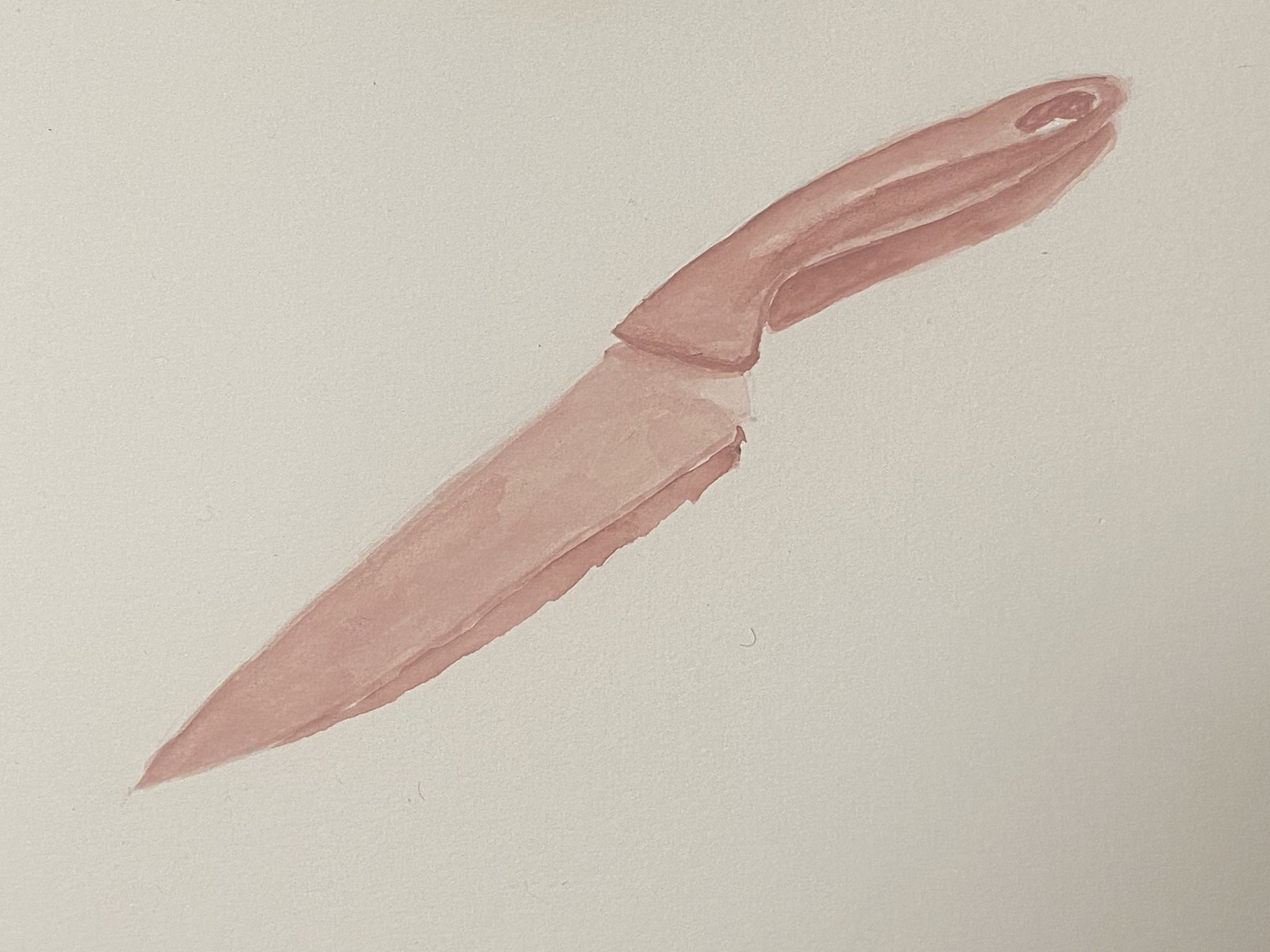This illustration is a delicate watercolor sketch depicting a knife, rendered in soft, muted shades of brownish pink against a cream-colored background. The composition places the blade diagonally, angling towards the lower left-hand corner, while the handle extends upwards to the upper right-hand corner. Though the image lacks intricate details, there is a subtle use of depth and shadow that gives the knife a tangible presence. The blade features a noticeable curve along its right edge, tapering to a sharp, defined tip. The handle is simplistic, marked by an oval hole near its top, adding a touch of realism to this otherwise minimalist artwork.